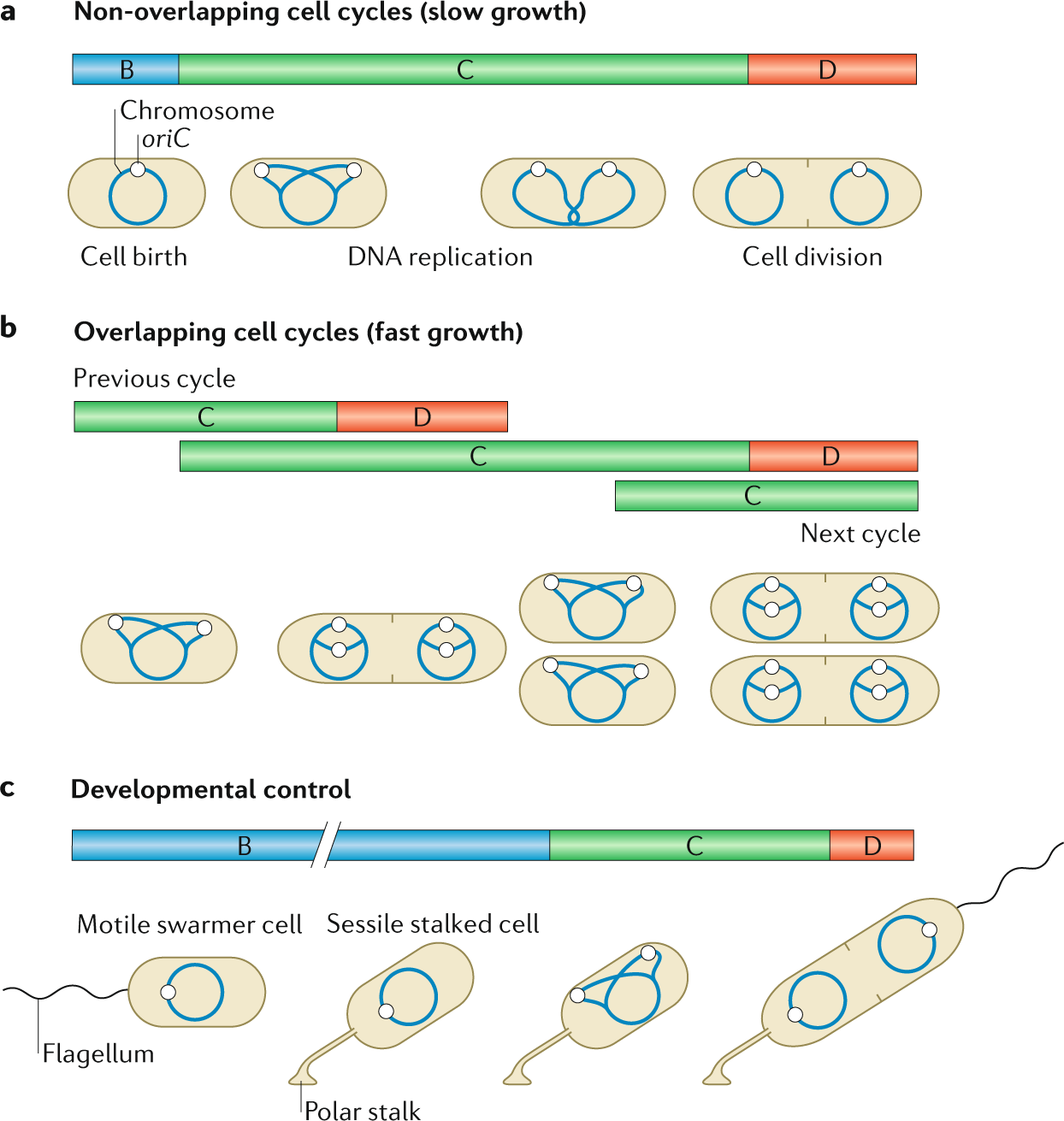This detailed color diagram, resembling a page from a biology textbook or a scientific poster, is divided into three main sections labeled A, B, and C. At the top, section A, titled "Non-overlapping Cell Cycles, Slow Growth," illustrates stages such as cell birth, DNA replication, and cell division, highlighted by a blue background and issuing labels B, C, and D over corresponding areas shaded blue, green, and orangey-red, respectively. Section B, titled "Overlapping Cell Cycles, Fast Growth," utilizes tan-colored, pill-shaped ovals with chromosomal illustrations to contrast the previous and next cell cycles, emphasizing rapid growth with overlapping cycles. The final part, section C, labeled "Developmental Control," depicts various cellular stages and structures, including motile swarmer cells equipped with flagella, sessile stalk cells, and polar stalks, which are represented with gray, blue, and black coloration. This comprehensive diagram effectively demonstrates the differences in cellular growth and development processes.